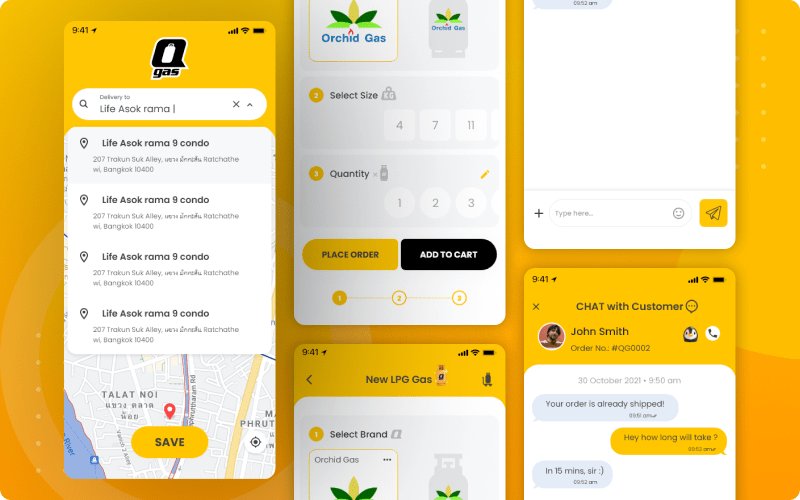Here is a detailed and cleaned-up descriptive caption for the image:

---

The image consists of five smartphone screenshots displayed side by side. 

**First Screenshot (Far Left):**
- The screen is a gas delivery interface titled "Delivery 2," located at "Life Asok Rama 9 Condo." 
- There are four location icons indicating multiple addresses within the same complex. 
- A Google Map preview is present with a "Save" button and an additional location icon.

**Second Screenshot (Top Middle):**
- This screen displays the "Orchid Gas" selection interface.
- Below the title, there is a drop-down box for selecting sizes: 4, 7, and 11 liters.
- Another box below allows users to specify the quantity: 1, 2, or 3 units.
- There are two buttons at the bottom: a yellow placeholder button and a black "Add to Cart" button.
- Three bubbles numbered "1," "2," and "3" indicate steps in a process.
- The current selection is highlighted as "Orchid Gas."

**Third Screenshot:**
- This screenshot shows the "New LPG Gas" selection interface.
- A gray box allows the user to select the gas brand, with "Orchid Gas" currently selected.
- Standard interface icons are visible at the top, including a timestamp (9:41), a send icon, Wi-Fi icon, and a half-full battery icon.

**Fourth Screenshot:**
- This screen is a chat interface, with half of it appearing empty.
- At the bottom, there are options to type a message, select emojis, and press a send button.
- Standard interface icons (timestamp, send icon, Wi-Fi icon, battery icon) are present.

**Fifth Screenshot (Far Right):**
- Another chat interface with the same standard icons.
- The chat history shows a conversation with a customer named John Smith.
- Order details include an order number, a photograph of John Smith, and the date "30 October 2021 at 9:50 PM."
- A gray message box indicates the order has already shipped.
- John Smith's response asks about the delivery time, to which a follow-up message states it will take "15 minutes, sir."

---

This caption provides a comprehensive overview of the contents and structure of each screenshot in the image.